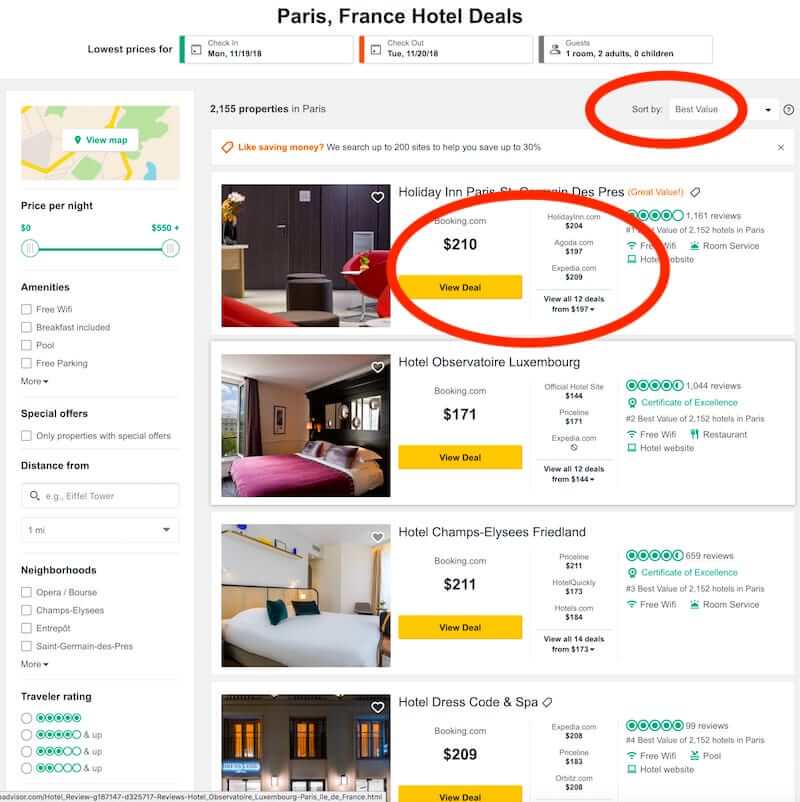**Screenshot Description of Paris, France Hotel Deals Webpage**

The screenshot depicts a webpage presenting hotel deals in Paris, France, organized under a well-structured layout with various filters and search options. Below is a detailed breakdown of the elements described:

1. **Heading and Date Selection:**
   - **Heading:** "Paris, France Hotel Deals"
   - **Date Selection:**
     - **Check-in:** *Monday, 11/19/18*, marked by a green vertical bar and accompanied by a calendar icon.
     - **Check-out:** *Tuesday, 11/20/18*, marked by a red vertical bar with a calendar icon.

2. **Guest Information:**
   - A gray vertical bar with icons depicting two persons (one darker and one lighter shade) labeled "Guests."
   - **Details:** 1 room, 2 adults, 0 children.

3. **Filter Options:**
   - **Price per Night:** "$0 to $550+" with a sliding scale.
   - **Amenities:** 
     - *Free Wi-Fi, Breakfast included, Pool, Free Parking* with corresponding checkboxes.
     - "More" option with a down arrow.
   - **Special Offers:** Checkbox for "Only properties with special offers."
   - **Distance From:** Search box with magnifying glass icon and a dropdown for selecting distance (initially set to "1 mile").
   - **Neighborhoods:** 
     - *Opera/Bourse, Champs-Elysées, Enfants Rouges, Saint-Germain-des-Prés* with checkboxes.
     - "More" option with a down arrow.
   - **Traveler Rating:** 
     - Filter by circles (rating levels from 2 to 5 and up).

4. **Main Content Area:**
   - **Total Properties Listed:** 2,155 properties in Paris.
   - **Sort Option:** Dropdown titled "Sort by" with a default value "Best value," enclosed in a red oval.
   - **Promotional Banner:** Features a golden ticket icon with the text, "Like saving money? We search up to 200 sites to help you save up to 30%.", and an "X" to close on the right.

5. **Highlighted Hotel Deals:**
   - **Hotel 1: Holiday Inn Paris Saint-Germain-des-Prés**
     - *Label:* "Great value" indicated in gold.
     - *Image:* Dark wood door, closets, black footstools, red chairs, a table, and a podium.
     - *Prices:*
       - Booking.com: $210 (highlighted in yellow as a view deal button).
       - HolidayInn.com: $204.
       - Agoda.com: $197.
       - Expedia.com: $209.
       - "View all 12 deals from $197" link.
     - *Rating:* 4 circles out of 5 from 1,161 reviews.
     - *Amenities:* Free Wi-Fi, room service.
     - *Highlight:* A red oval around the deal details.
   - **Hotel 2: Hotel Observatoire Luxembourg**
     - *Image:* Bed with a maroon cover, silky pillowcases, black headboard with mirrors, off-white picture, dark carpet and curtains, open windows with exterior views.
     - *Prices:*
       - Booking.com: $171.
       - Official Hotel Site: $144.
       - Priceline: $171.
       - "View all 12 deals from $144" link.
     - *Rating:* 4.2 circles out of 5 from 1,044 reviews.
     - *Label:* Certificate of Excellence, 2nd best value.
     - *Amenities:* Free Wi-Fi, restaurant.
   - **Hotel 3: Hotel Champs Elysees Freland**
     - *Image:* Bed with white linens, black pillowcases, wooden headboard, shelf with blue and yellow items, off-white walls, and yellowish drapery.
     - *Prices:*
       - Booking.com: $211.
       - Priceline: $211.
       - HotelQuickly: $173.
       - Hotels.com: $184.
       - "View all 14 deals from $173" link.
     - *Rating:* 4.2 circles out of 5 from 659 reviews.
     - *Label:* Certificate of Excellence, 3rd best value.
     - *Amenities:* Free Wi-Fi, room service.
   - **Hotel 4: Hotel Dress and Code Spa**
     - *Image:* Exterior view of a building with brick or stone facade showing three windows with light behind them, including a door with white light.
     - *Prices:*
       - Booking.com: $209.
       - Expedia.com: $208.
       - Priceline: $183.
       - Orbis.com: $208.
     - *Rating:* 5 circles out of 5 from 99 reviews.
     - *Label:* 4th best value.
     - *Amenities:* Free Wi-Fi, pool.

This detailed summary provides a comprehensive understanding of the elements and information presented in the screenshot of the hotel deals page for Paris, France.